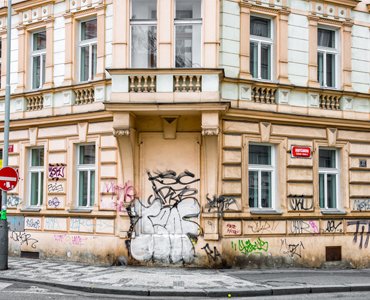The photograph depicts an elegant, old two-story building, showcasing European architectural stylings with its ornate and detailed features. The facade is painted in white with cream-colored window decorations and intricate filigree detailing above each window. A notable feature of the building is a pair of double doors on the second floor that open onto a small balcony. 

However, the beauty of this building is marred by graffiti. The street-facing sides of the building, situated at a corner with a rounded sidewalk, are covered in graffiti. The most prominent piece is a large, elaborately done tag in white and black with circular, curvy letters, positioned prominently at the building's corner on ground level. Smaller, simpler tags and signatures, using a single color, scatter around this central tag. A lamppost stands on the sidewalk near the building, and the scene includes part of the surrounding street.